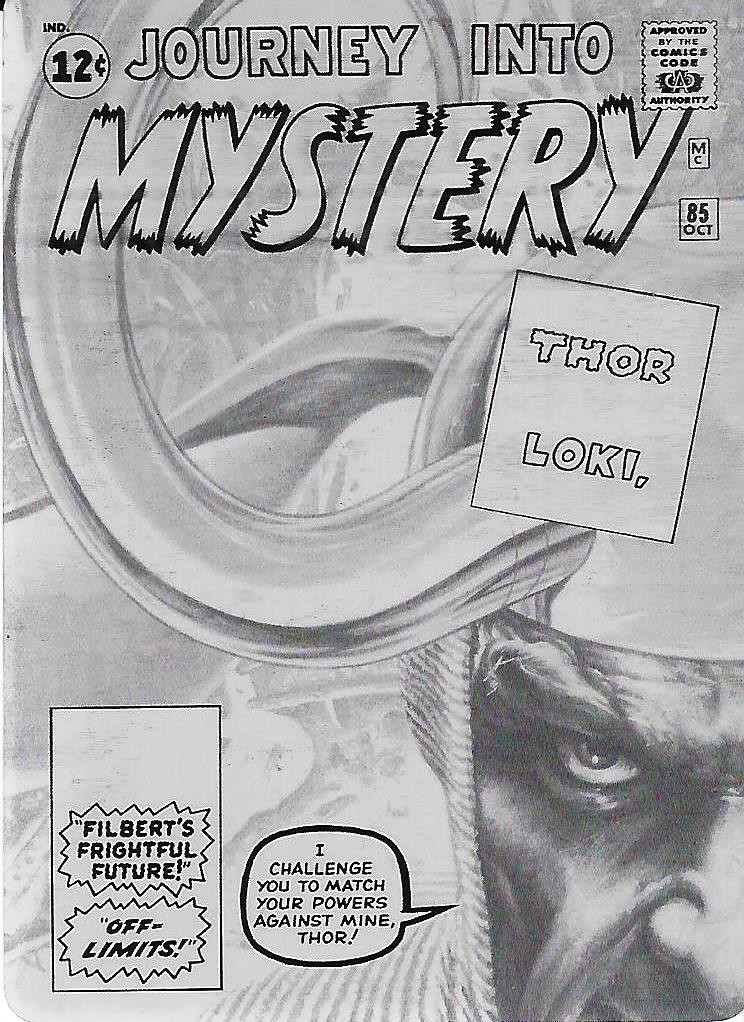The black-and-white comic book cover features a stylized title at the top, "Journey into Mystery," with the word "Mystery" prominently displayed in a large, stylized font. In the upper left corner, there is a small circle containing the price, "12 cents," while the upper right corner bears a stamp-like image that reads "Approved by the Comics Code Authority" and the date "MC 85 October." Below the title, a square box contains the names "Thor" and "Loki." 

Dominating the cover is a detailed pencil drawing of Loki, identifiable by his horned helmet. Loki has an angry expression and is depicted speaking through a speech bubble that says, "I challenge you to match your powers against mine, Thor." Additionally, a small white box in the left corner advertises another story titled "Philbert's Frightful Future, Off Limits." The entire layout, including the borders of the text boxes, is rendered in black and white.